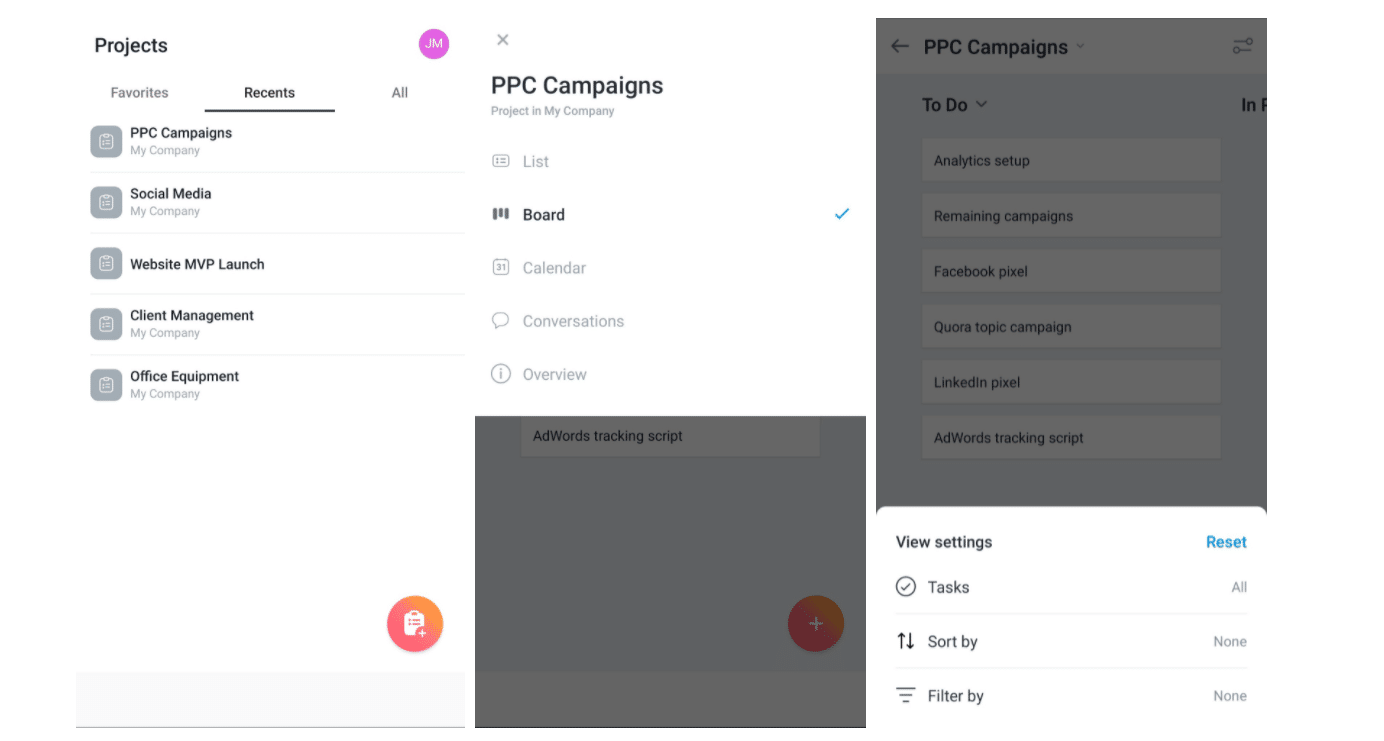Caption: 
The image series consists of screen captures showcasing an organizational interface, likely from a project management tool with a clean, minimalistic design.

1. **First Image:**
   - The background features a stark white backdrop with predominantly black text.
   - A distinct purple and white circular icon adds a splash of color.
   - The title "Top Black Projects" is prominently displayed.
   - It is divided into three categories: "Favorites," "Recents," and "All," with a black line beneath the "Recents" tab to indicate the active section.
   - A list of project names each accompanied by gray icons includes: "PPC campaigns," "Social Media," "Website MVP Launch," "Client Management," and "Office Equipment."
   - An orange circle with a white price tag icon is positioned at the bottom, perhaps representing an actionable button.

2. **Second Image:**
   - The top section includes a gray "X" for closing the pop-up.
   - The title "PPC Campaigns, Project in my company" stands out in bold black text on a white background.
   - Below, various navigational options are displayed with icons:
     - "List" with a board icon and three horizontal lines.
     - "Calendar" with a calendar icon.
     - "Conversations" featuring a speech bubble icon.
     - "Overview" marked by an eye encased in a circle icon.
   - A gray box contains an orange and white circular icon with the label "AdWords Tracking Script."

3. **Third Image:**
   - The background is gray, listing tasks under "PPC Campaigns To-Do."
   - Each task is a white box with black text:
     - "Analytics Setup"
     - "Remaining Campaigns"
     - "Facebook Pixel"
     - "Quora Topic Campaign"
     - "LinkedIn Pixel"
     - "AdWords Tracking Script"

4. **Fourth Image:**
   - Features a white box with black text.
   - Includes the term "Reset" in blue, suggesting a clickable option.
   - The phrase "View Settings Task" is displayed alongside a circular icon with a check mark.
   - Options listed include:
     - "Task All" 
     - "Sort by None" with an adjacent up-and-down arrow.
     - "Filter by None" with a funnel icon.

Overall, the images exhibit a highly organized and intuitive project management interface delineating categories, tasks, and settings with clear iconography and a minimalist aesthetic.